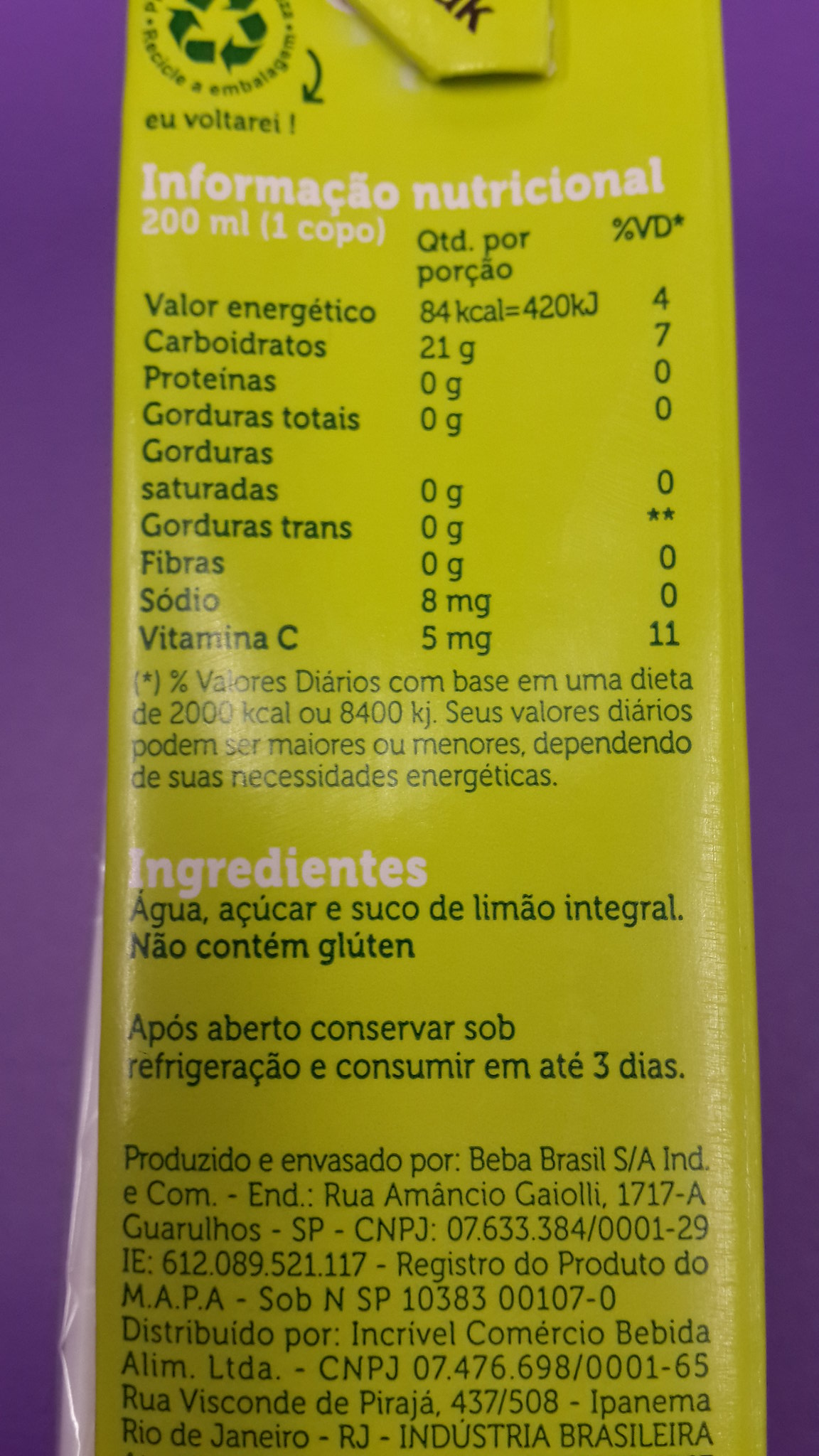The image depicts a nutritional label on a carton, primarily in a language that appears to be Spanish. Several nutritional components are recognizable, including proteins, saturated fats, sodium, and vitamin C. The list of ingredients begins with "aqua," which translates to water. The carton itself is partially visible on the lower left side of the image, with its white front face in view. The label is set against a purple background, and it is predominantly lime green. The text on the label is either black or white, with white being used for the headlines. Additionally, there is a recycle symbol present on the label, and this, too, is in a different language.